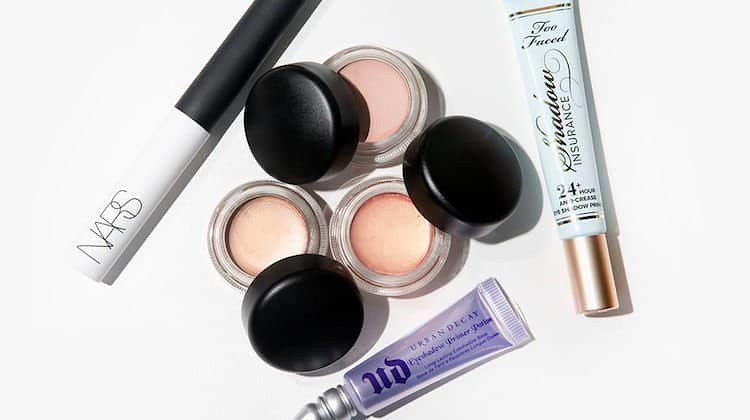The image showcases a selection of various high-quality makeup products arranged on a pristine white background. Prominently displayed is a white tube with a black lid labeled "NARS." Central to the photograph are three elegant glass vials with black lids, aligned slightly askew. These vials likely contain highlighter, cream eyeshadow, blush, or similar products. To the side of these vials is a tube labeled "Too Faced Shadow Insurance," a renowned 24-hour eyeshadow primer. Near the bottom of the image, a small purple tube, identified as an eyeshadow primer from Urban Decay, is placed horizontally. This collection of sophisticated makeup products underscores both their aesthetic appeal and their functional diversity.